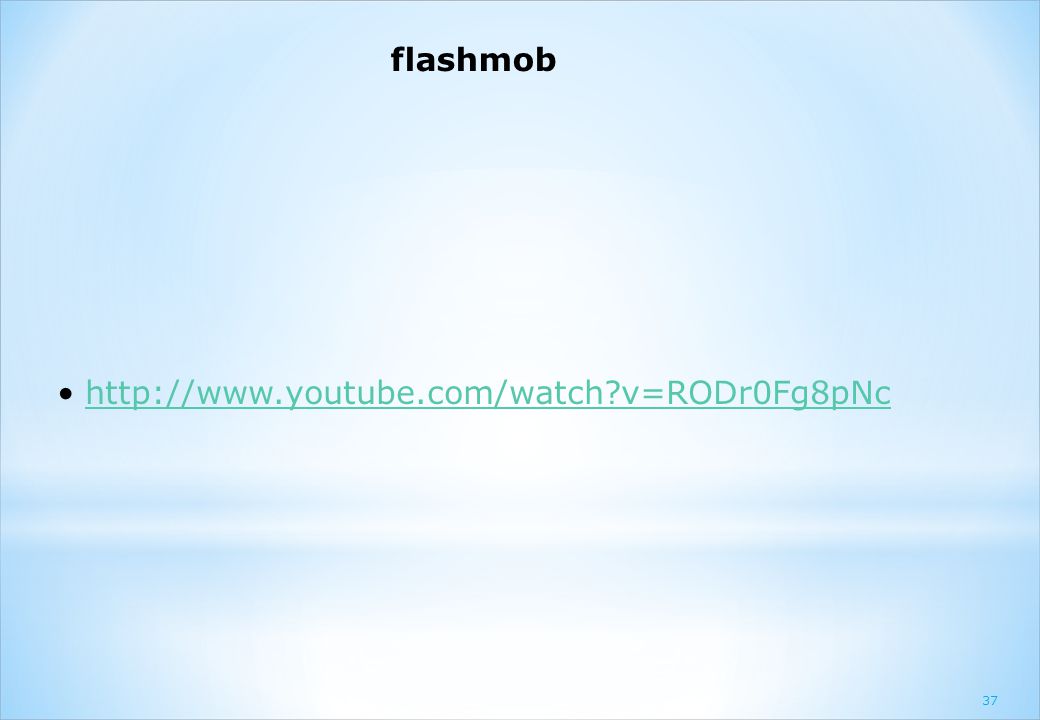The image is a screenshot resembling a PowerPoint slide with a minimalist design. The background is a light blue, creating a clean and simple visual. At the very top center, in small black lowercase font, the text "flash mob" is displayed. Beneath this, centrally aligned both horizontally and vertically, a single black bullet point is present. This bullet point is accompanied by a hyperlink which reads: "http://www.youtube.com/watch?v=RODr0FG8PNC". In the bottom right corner of the slide, the number "37" is noted, possibly indicating the slide number within a presentation. The overall layout suggests that this slide is part of a company's presentation, showcasing a direct link to a YouTube video related to a flash mob. The clear link and professional structure imply it could be used for educational or corporate purposes.